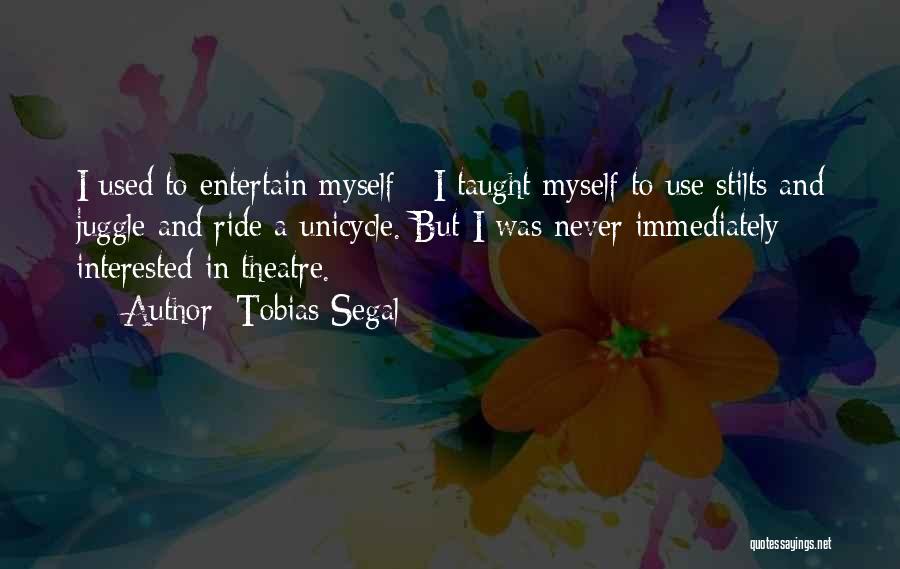The image appears to be a quote card with a pastel-colored background featuring shades of greens and blues, adorned with various blue curves and paint-like color slashes that artistically frame the text. The most prominent detail is an orange flower with a green center located towards the right center of the card. The quotation at the heart of the card, written in white, almost paint-like text, reads: "I used to entertain myself, I taught myself to use stilts and juggle and ride a unicycle, but I was never immediately interested in theater." This quote is attributed to Tobias Siegel, with his name positioned just below the text. In the bottom right corner, in smaller print, the source "quotesayings.net" is noted. The overall design, with its faded dark grey elements and detailed font, highlights the text against the pastel and floral background.